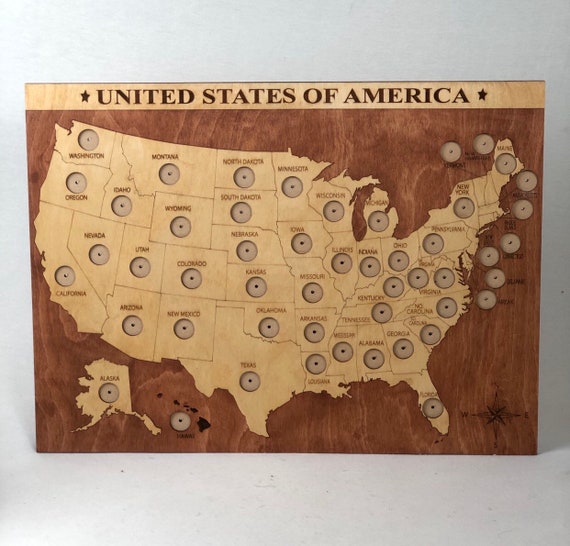The image depicts a vertically rectangular wooden board with a polished dark wood background and a lighter wood overlay forming a detailed map of the United States. The map showcases all the states in a light brown shade, each labeled with its respective name. Every state has a small circular hole in its center, designed to hold a commemorative quarter. At the top of the board, a horizontal strip in light brown wood prominently features the inscription "UNITED STATES OF AMERICA" in capital letters. The entire setup appears to be staged indoors with artificial lighting, casting a noticeable shade along the right side and a lighter spot in the upper left corner of the grey background. This board seems to be a collector's piece for displaying the state quarters released some years ago.